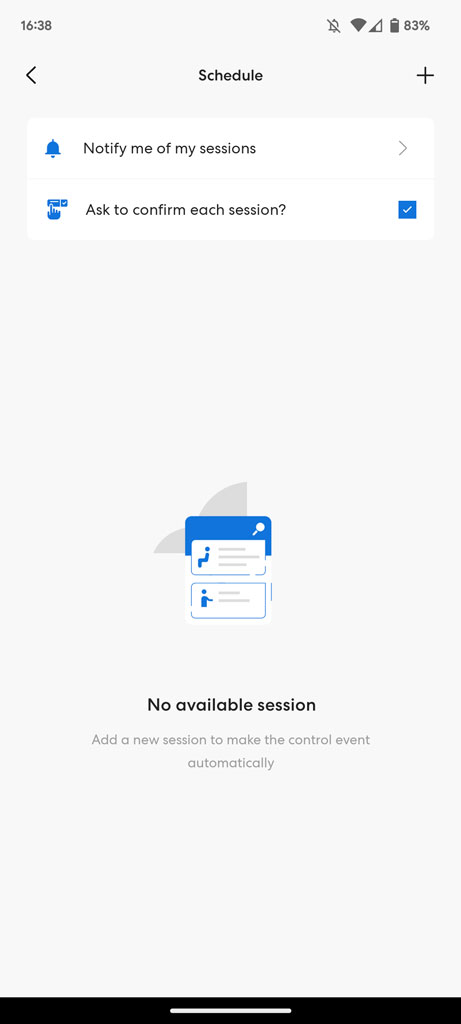This vertically rectangular image showcases a screenshot from a cell phone with a predominantly gray background and a thin black horizontal banner at the bottom. At the top of the screen, the current time displayed is 16:38. The status bar on the upper right corner features various icons: an alarm off symbol, Wi-Fi connectivity, cellular signal strength bars, and a battery icon indicating 83% charge.

Central to the screen is the heading "Schedule," flanked by a back arrow on the left and a plus sign on the right. Directly below "Schedule," the text "Notify me of my sessions" is followed by a checked option to "Ask to confirm each session." Further down, an icon representing a session is visible.

The main body of the screen displays the text "No available session" in black. Below this, in gray text, is the instruction, "Add a new session to make the control event automatically." This detailed layout highlights the functionality related to managing sessions on the device.